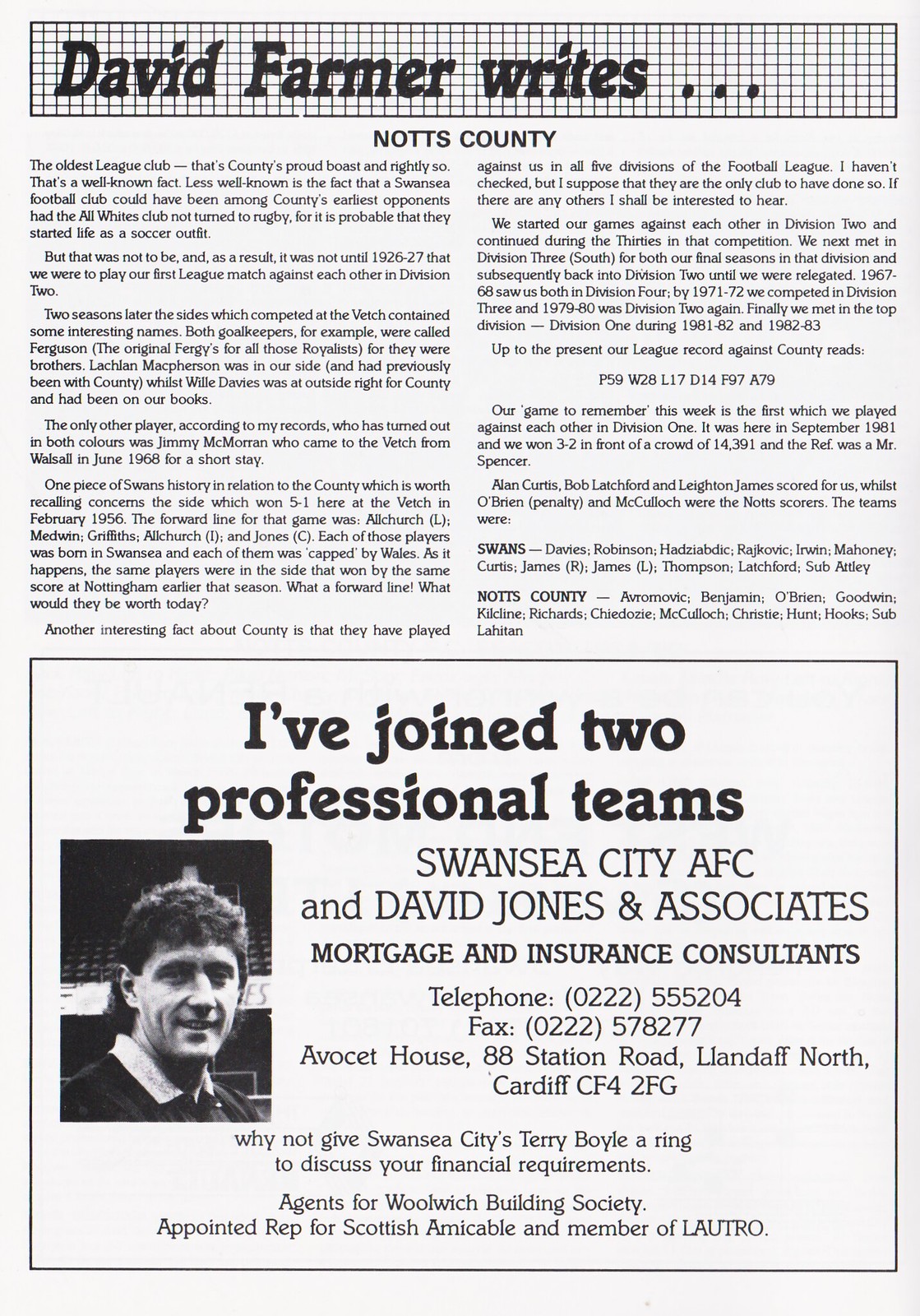The image depicts a page from a magazine or pamphlet set in the United Kingdom, featuring both an article and an advertisement. The page is titled "David Farmer Writes..." with a subtitle that reads "Notts County." The article begins with a historic note about Notts County, highlighting its status as the oldest league club, and exploring a lesser-known fact about Swansea Football Club's early days in soccer before switching to rugby. The textual content spans two columns and extends across the upper part of the page.

The lower half of the page is dominated by an advertisement blending professional football and financial services. The ad states, "I've joined two professional teams, Swansea City AFC and David Jones and Associates, mortgage and insurance consultants." There is a black-and-white profile photo of who appears to be a soccer player, located in the lower left corner. The ad features the invitation, "Why not give Swansea City's Terry Boyle a ring to discuss your financial requirements?" and lists affiliations with Woolwich Building Society, Scottish Amicable, and LAUTRO.

The page has a white background with predominantly black text. The image of the man, identified as Terry Boyle, integrates seamlessly into the design, providing a visual anchor in the lower section of the page. The layout and content collectively speak to the reader's interests in both football and financial planning services.